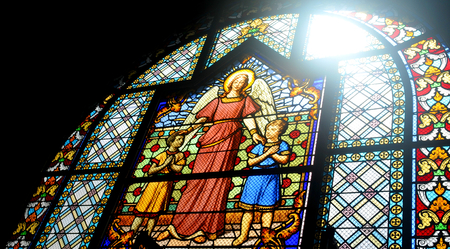The image features a stunning arched stained glass window commonly seen in churches. The primary focus is a central rectangular panel topped with a triangular arch, depicting an angel with a yellow halo, adorned in long red robes and white wings. The angel, radiating grace, reaches out to two children: their left hand touches the head of a black-haired child with slightly darker skin, dressed in orange, while the right hand rests on the shoulder of a blond-haired, lighter-skinned child in blue. This holy scene is set against a decorative backdrop of green circles with red dots and white, rock-like formations. A black, pentagon-shaped border frames this central tableau, which contrasts with the sunlit upper corners. Surrounding the main panel is a standard stained glass pattern of white diamonds, blue and yellow lines, and small orange or yellow spots. The outermost edge is adorned with a vibrant border resembling a royal, ornately decorated banner in red, white, and yellow hues.